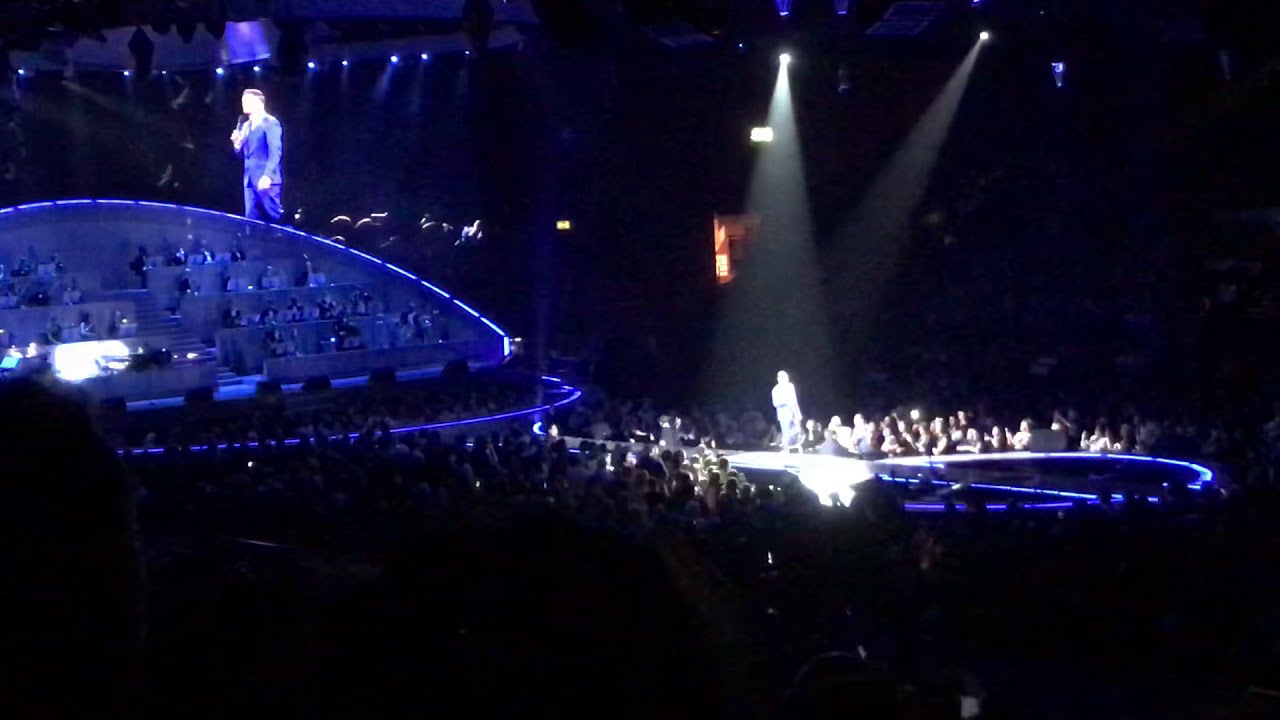The image depicts a large, dimly-lit concert hall or auditorium filled with a substantial crowd. Central to the scene is a performer, possibly a singer or a speaker, dressed in a blue or purple suit and holding a microphone. He stands on an oval-shaped stage that extends into the audience, illuminated by a spotlight. The stage and surrounding area are accented with vivid blue and purple LED lights, casting a dramatic ambiance. In the background, there is a sizeable video screen displaying an enlarged image of the performer, suggesting it's there to aid visibility for distant attendees. The audience is spread across both sides of the stage, with additional seating on elevated platforms and booths that might serve as VIP sections. The venue's ceiling features blue lights and several white cones of light streaming downward, adding to the overall theatrical atmosphere. The heads of audience members in the foreground appear larger, indicating the viewer's proximity to this crowd, while those further away become indistinct amidst the vast sea of attendees.